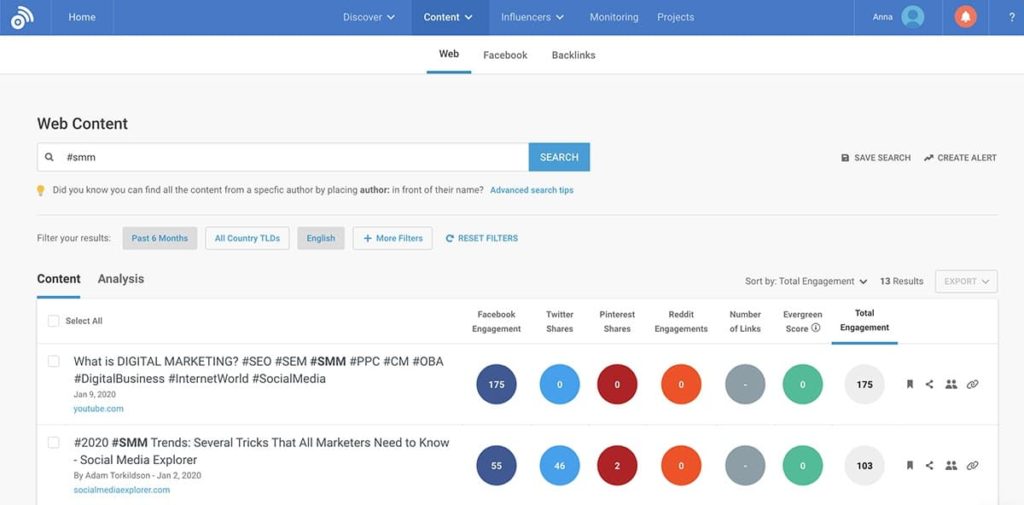A detailed screenshot of a user interface, showing a webpage design with a prominent blue border running across the top. In the top-left corner, the label "Home" is visible. Spanning across the top are the following menu items: "Discover," "Content," "Influencers," "Monitoring," and "Projects." The top-right corner features the user name "Anna" beside a circular icon depicting a person, followed by another circle with a red background containing a white bell icon, indicative of notifications. Farther to the right, there is a question mark icon.

Below this header section, the text "Web Facebook Backlinks" is displayed. Further down, it reads "Web Content," followed by a search bar situated on the left with a magnifying glass icon. The search bar contains the text "#SMM" and has the word "Search" positioned on the far right side.

The interface also provides a helpful suggestion that reads: "Did you know that you can find all the content from a specific author by placing ‘author:’ in front of their name? Advanced Search Tips." Adjacent to this is a section offering filtering options with the prompts: "Filter your results: Past six months, all country TLDs, English" along with an option for "More filters" and a button labeled "Reset Filters."

The main content area below this includes two columns: "Content" and "Analysis." It offers selection options such as "Select All" for metrics like "Facebook Engagement," "Twitter Shares," "Pinterest Shares," "Reddit Engagements," "Number of Links," "Evergreen Score," and "Total Engagement."

Underneath these options, there is an example article titled "What is Digital Marketing?" accompanied by various hashtags such as "#SEO," "#SEM," and "#PPC," along with additional text and symbols decorating the page.